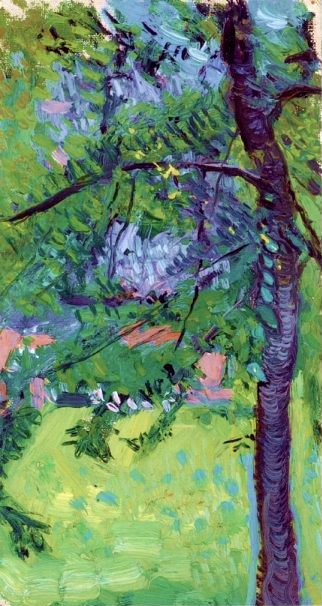The image is a detailed hand-painted artwork depicting an outdoor scene, likely set in the middle of the day. The focal point of the painting is a tall and narrow tree trunk situated on the right side of the image, extending vertically from the bottom right toward the top. Branches protrude from the tree toward the center and left side, adorned with numerous green leaves. Perched on these branches are various small black and white birds. The ground is covered in light green grass, interspersed with blue flowers, creating a lush foreground. In the background, a grey mountain looms, providing a natural backdrop for several brown houses nestled at its base. The colors in this painting are a harmonious blend of greens, blues, browns, and grays, with the branches exhibiting a grayish-purplish brown hue. The painting's style suggests it is an oil painting, possibly intended for display in an art exhibition.